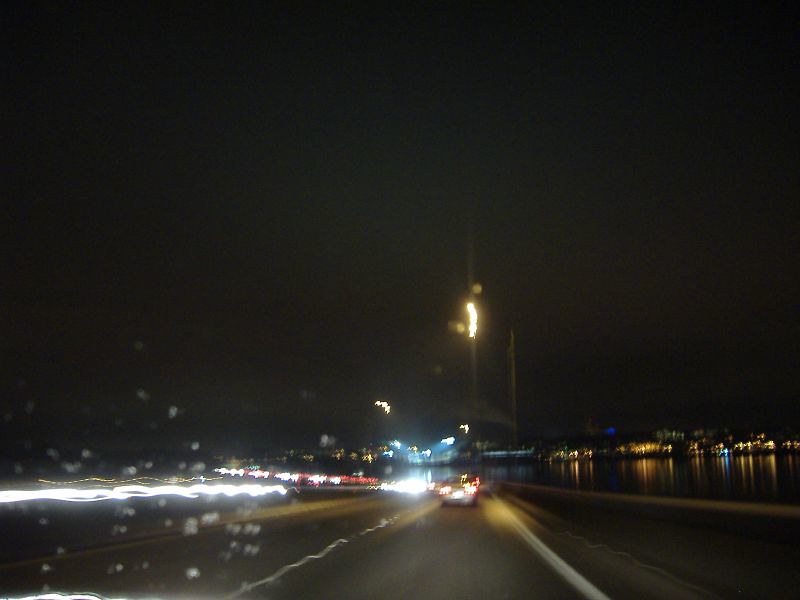The image captures a nighttime scene illuminated by the headlights of a moving vehicle, likely taken from a dashcam mounted on the front windshield. Raindrops are splattered across the glass, indicating it’s raining. The scene is somewhat blurry, perhaps due to the vehicle's motion combined with the precipitation. The wet, possibly reflective road is clear immediately around the vehicle, but several cars are lined up ahead, suggesting the onset of a traffic jam. To the right of the street, a body of water—either a river or a lake—runs parallel, providing a serene contrast. Across the shoreline, the lights of numerous buildings twinkle, adding an urban glow to the dark scene. Various yellow-white street lamps, perched atop poles along the right side of the road, further illuminate this rainy, urban landscape.